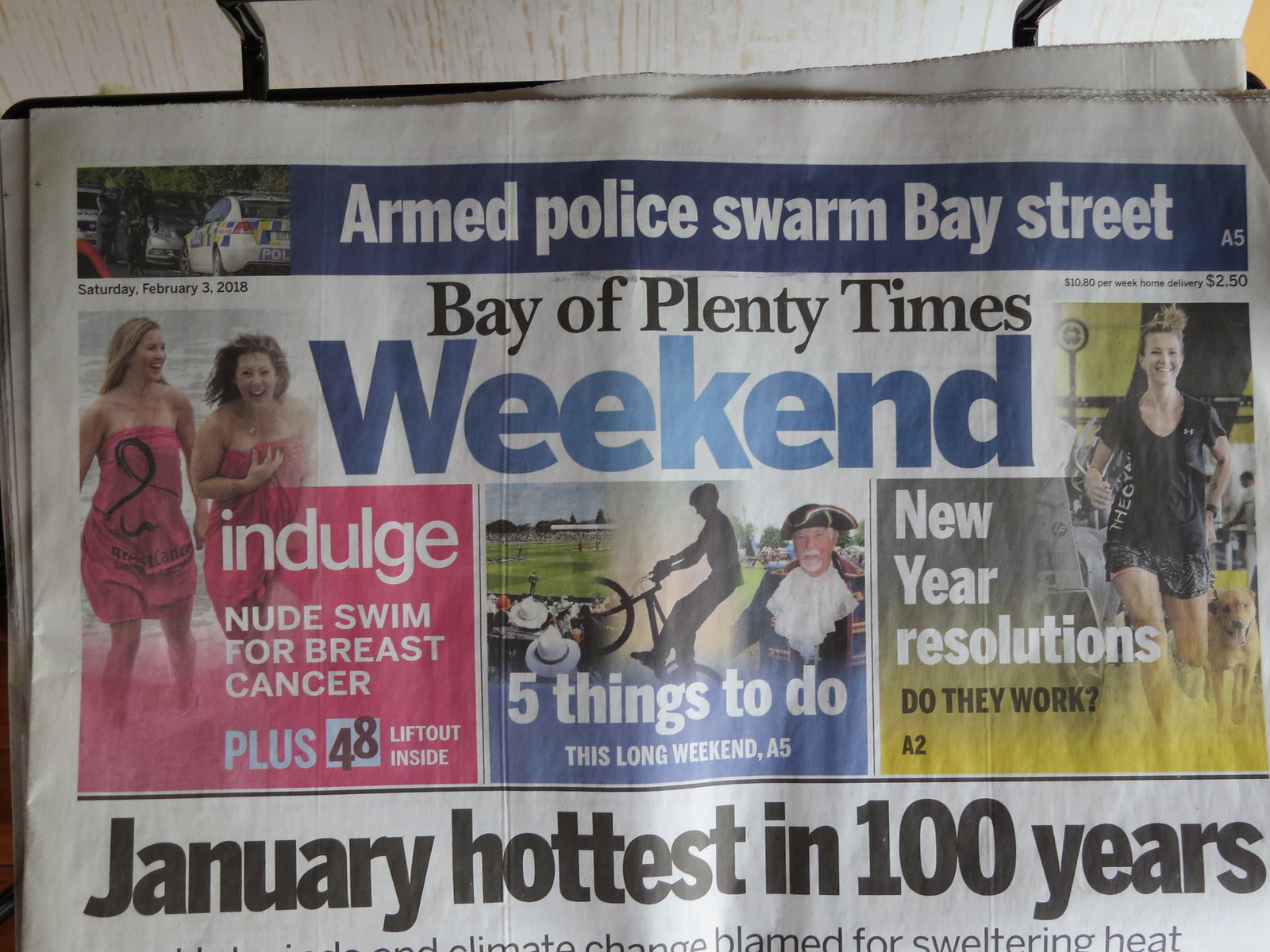The photograph captures the top half of a white newspaper page filled with multi-colored text and images. Dominating the top is a blue horizontal banner with white text proclaiming "Armed Police Swarm Bay Street," accompanied by a small image of a police vehicle on a street to the left. Additionally, the banner notes "A5" on the lower right, with "Saturday, February 3rd, 2018" and subscription details "$10.80 per week home delivery, $2.50" beneath it.

Center-aligned, the heading "Bay of Plenty Times" is displayed in bold black text, with the word "Weekend" in large blue letters beneath it. The main content features three photographs arrayed horizontally:

1. On the left, two Caucasian women enjoy a beach wrapped in pink towels, with the caption "Indulge Nude Swim for Breast Cancer, plus $48 lift-out inside."
2. Centrally, a man dressed as a pirate stands next to a boy on a bicycle with a stadium in the backdrop, captioned "Five Things to Do This Long Weekend, A5."
3. To the right, a yellow-bordered image shows a woman running with her dog, captioned "New Year's Resolutions. Do They Work, A2."

Below these images, a headline in black text reads, "January Hottest in 100 Years, Climate Change Planned for Sweltering Heat." The composition suggests the setting is likely indoors, with the newspaper centered as if laid out on a table.